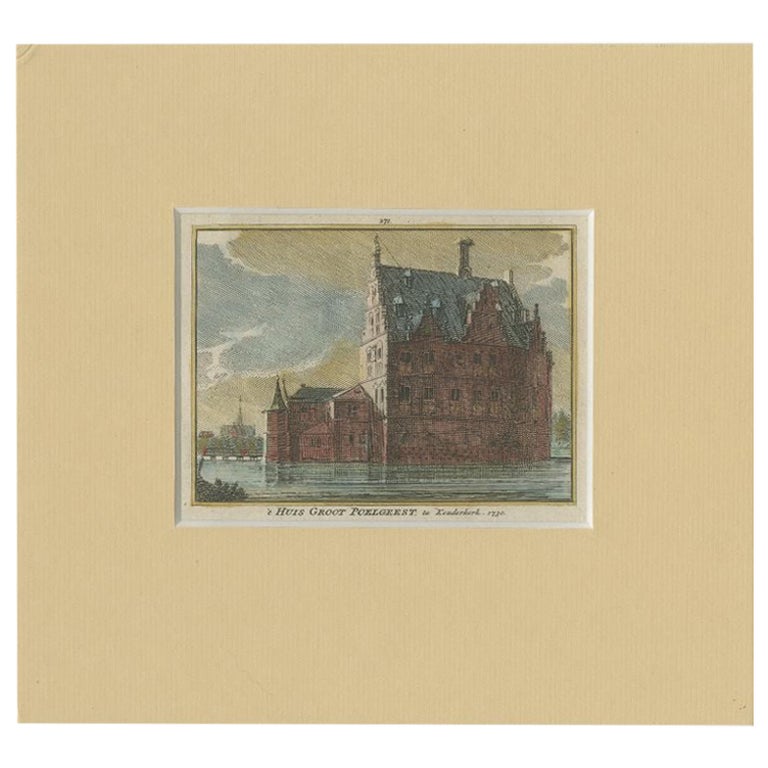A light mustard-colored frame encompasses the entirety of this image, emphasizing a contrast with the central brown-colored building. The building, which has a dark charcoal gray rooftop, stands prominently within the frame. Displayed on the building is text that reads "Hughes Route Pellegrini." Above the structure, gray clouds hover, adding a dynamic element to the scene. Additionally, parts of the building have noticeable beige tones, adding texture and depth to its appearance. The building's architecture features an intriguing asymmetry, appearing significantly larger on the right side compared to the smaller left side.